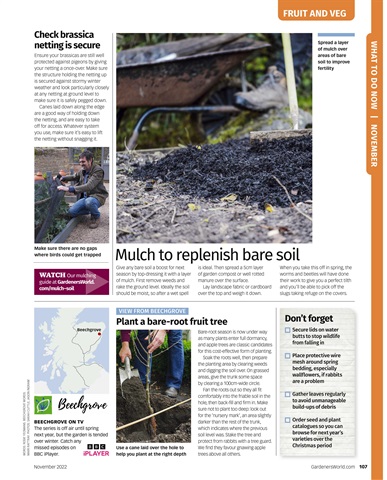This is a detailed description of a digital interface, possibly a website or an online magazine page dedicated to gardening, potentially named "GardnerWorld.com" indicated by text in the bottom right. The layout is reminiscent of a printed magazine. 

In the upper left corner, there's a noteworthy article advising gardeners to check that their brassica netting is secure, illustrated by an individual adjusting or inspecting nets in a modest garden setting. Adjacent to this piece is another article focused on the benefits of mulch for replenishing bare soil, accompanied by an image of rich, black mulch in a wheelbarrow, positioned on parched, brown soil. 

A navigational tab at the top of the page hints at an informative section dedicated to fruits and vegetables, specifically detailing tasks suitable for November. Lower on the left, there's a mention of "Beach Grove on TV," although its significance, whether a location or a show, remains unclear. This is echoed by a vignette showing a view from Beach Grove. Next to this is an instructional article on planting bare root fruit trees, portrayed by a person using a spade to plant a seedling in a large, ready-dug hole amidst soft brown dirt.

On the far right, an area titled "Don't Forget" lists four gardening to-dos, though the details are too minuscule to decipher. This column is accentuated by an orange bar running along the entire right edge, reinforcing the visual layout akin to a magazine spread.